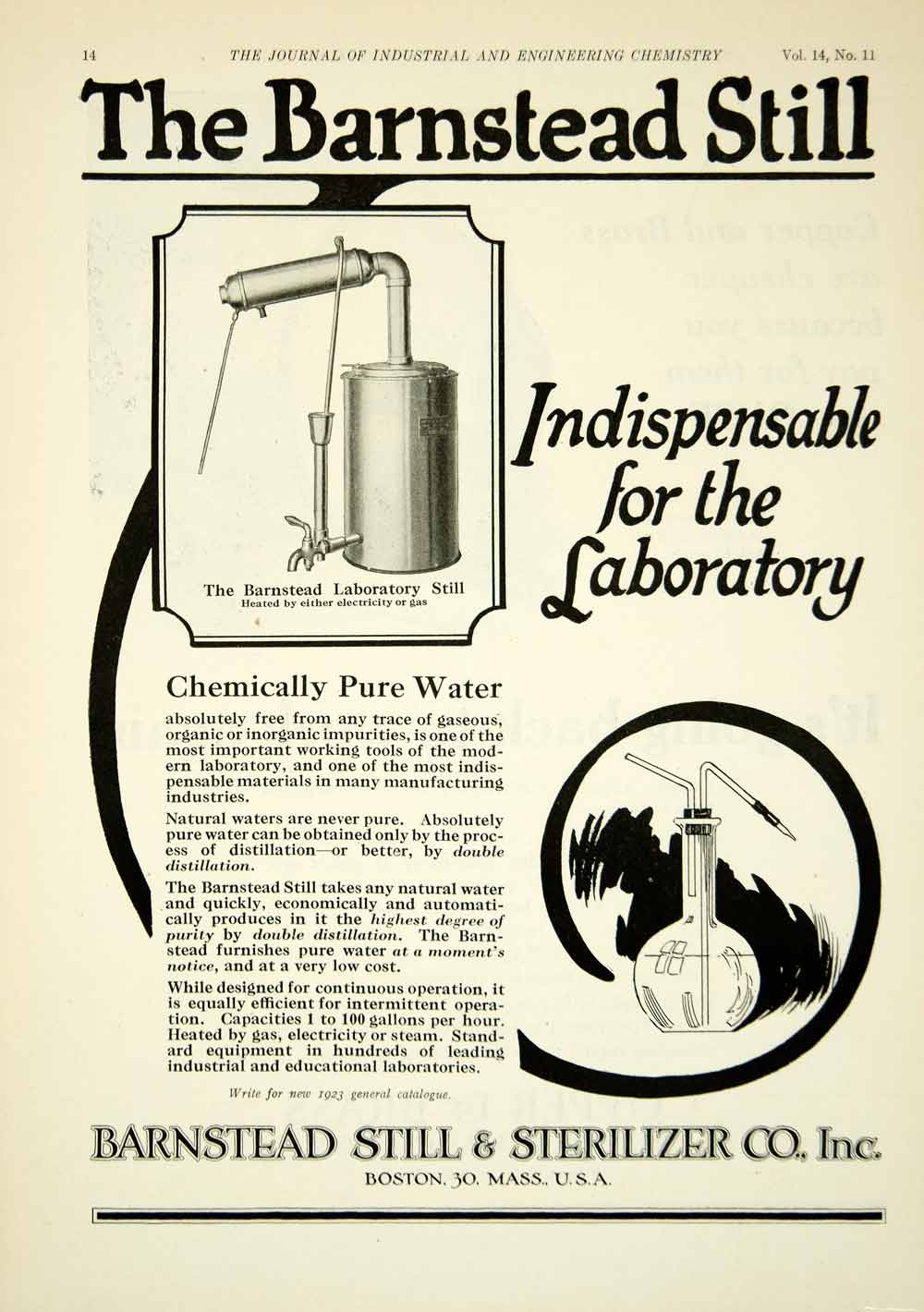The image depicts a vintage advertisement on an aged, yellowed page from the Journal of Industrial and Engineering Chemistry. At the top left corner is the page number 14, while the top right corner reads "Volume 14, No. 11". The title, "The Barnstead Still," is prominently displayed in bold and underlined, above a detailed illustration of the Barnstead Laboratory Still. This equipment is depicted as a rounded cylinder with a pipe extending upward and curving to the left, accompanied by a front tap, a longer pipe, and a small cup with a protruding pole.

Beneath the image, smaller text indicates the still can be heated by either electricity or gas, emphasizing its indispensability for laboratory use. Below this is the main article, which elaborates on the importance of chemically pure water in laboratories and manufacturing, explaining how the Barnstead Still efficiently produces such water through double distillation, with capacities ranging from one to 100 gallons per hour.

To the right of the image of the apparatus is another custom illustration of a conical beaker, featuring a cork with two glass tubes angled outwards, all set against a sketchy black background that resembles smoke. At the bottom of the page, small text invites readers to write for the new 1923 general catalog. The advertisement concludes with "Barnstead Still and Sterilizer Co., Inc." in bold text outlined in white, followed by the address "Boston. 30. Mass. U.S.A.," separated by a thin black line bordered in white.